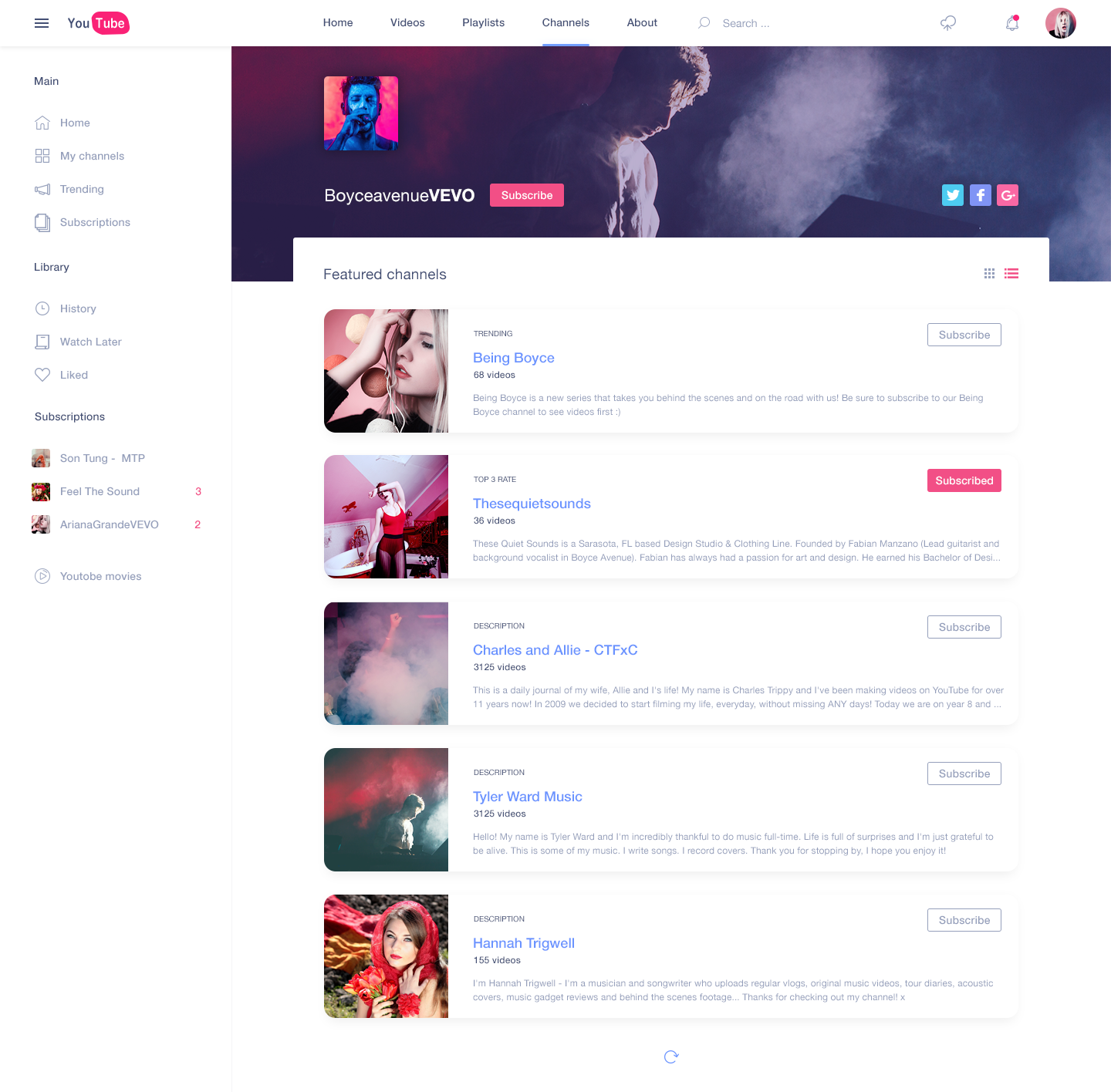This image is a YouTube screenshot from several years ago, as evidenced by the old YouTube logo. In the top left corner, the logo features "You" in black font and "Tube" in white font within a red box. The top menu displays options such as Home, Videos, Playlists, Channels, About, and a search box. The page in view is dedicated to a VEVO channel, specifically for an artist named "Boyce Avenue."

To the right, there is a red "Subscribe" button. The channel's header graphic depicts the artist in performance, surrounded by stage smoke from smoke machines, indicating a concert setting. On the left of this header, there is a stylized image where the artist's face is tinted blue against a pink background.

Below the header, there is a list of videos with thumbnails, but the small fonts make the titles hard to read. Among them, the first video is titled "Being Boyce Avenue," and the second one is "These Quiet Sounds." The section is labeled "Featured Channels," indicating that these are channels users can subscribe to.

On the left sidebar, various menu options are visible, including Home, My Channels, Trending, Subscriptions, Library, History, Watch Later, Liked videos, and Subscriptions again.